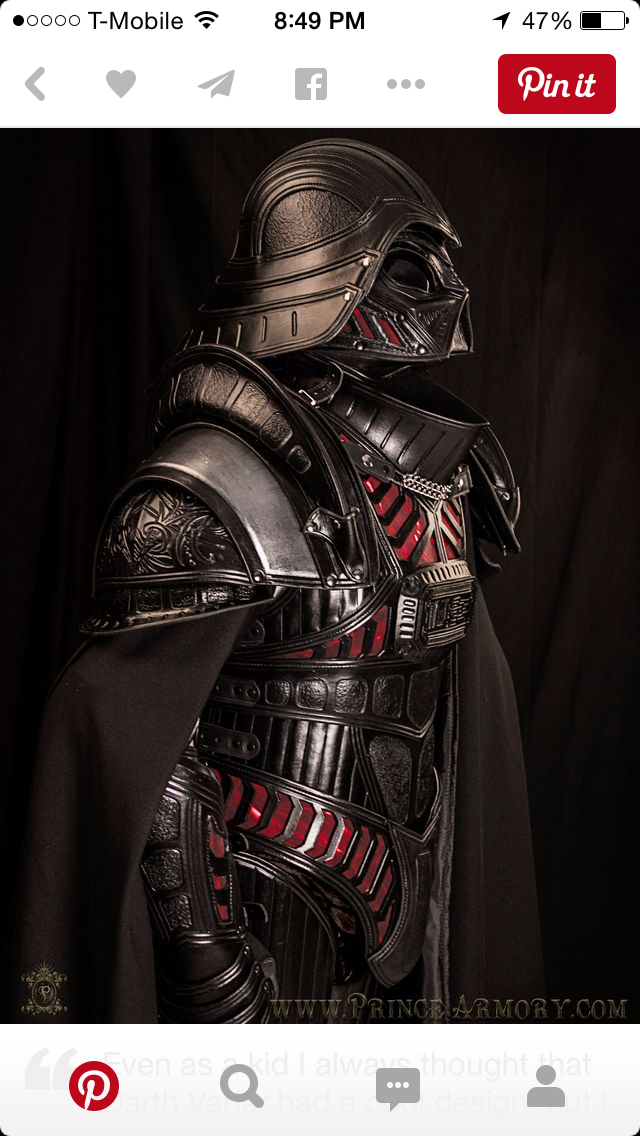This vertical rectangular image captures a mobile phone screenshot featuring a detailed view of a steampunk-inspired Darth Vader figure. The top of the screenshot displays standard mobile indicators: "T-Mobile" with a weaker Wi-Fi signal (one out of five circles filled), "8:49 PM" in the center, and a battery at 47% on the right. Directly below, the interface includes various icons: a left-pointing arrow, a heart, a paper airplane, a Facebook icon, an ellipsis, and a prominent red "Pin It" button against a white text background.

The primary focus of the image is a sideways view of what appears to be Darth Vader, wearing black armor accented with red steampunk elements on his torso, gauntlets, and mask, set against a black curtain backdrop. The text "www.princearmory.com" is faintly visible in the lower right-hand corner, suggesting the unique design's origin. The bottom portion of the screenshot features a light gray border with the Pinterest logo inside a red circle, a search icon, a comments icon, and a profile icon. Behind these icons, there is a slightly faded text in quotes saying, "I can see even as a kid I always thought that," which cuts off at the bottom.